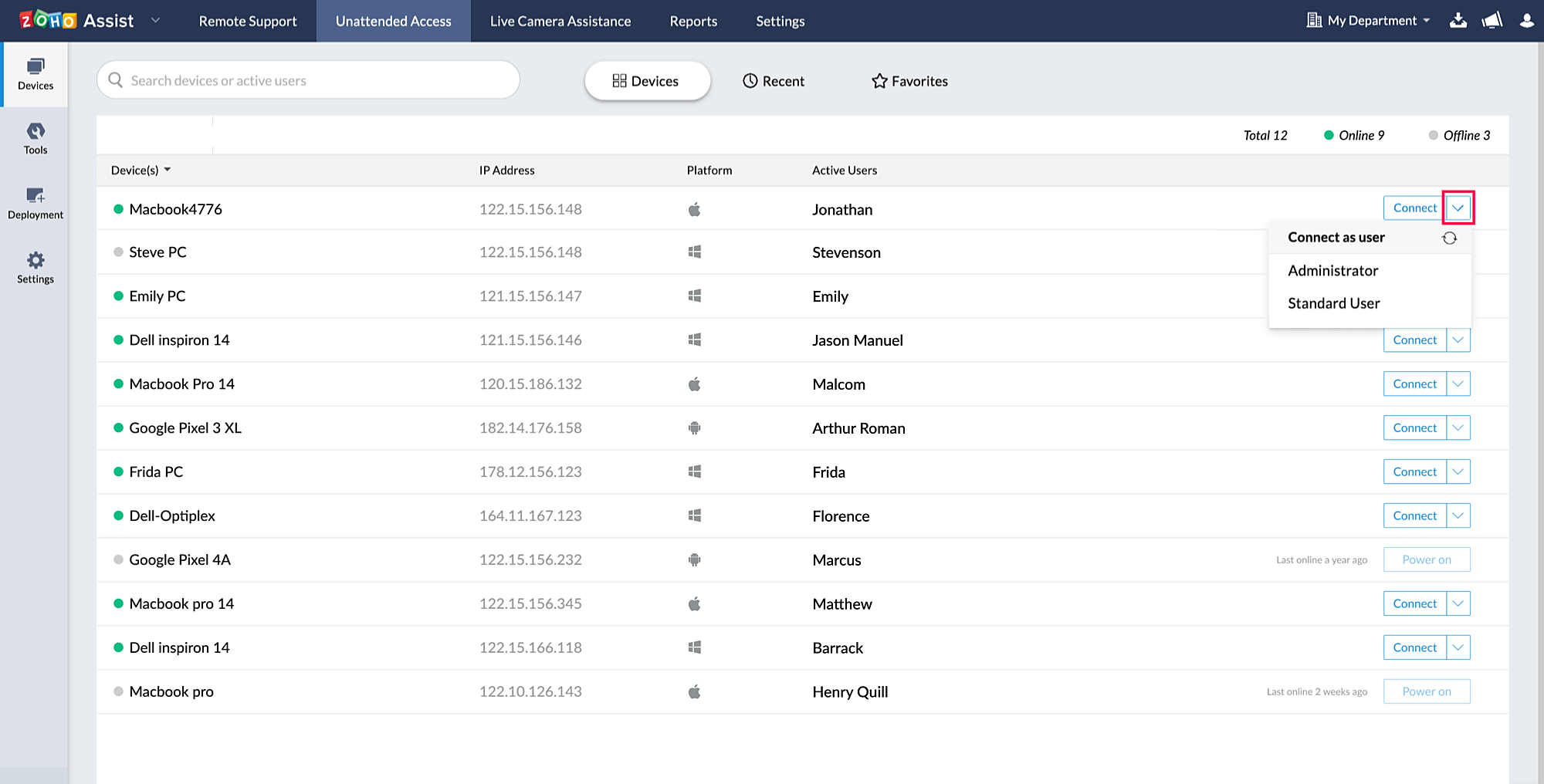A detailed screenshot of a website interface labeled "Zoho Assist." The title "Zoho Assist" appears prominently with each letter displayed on differently colored shapes or blocks in red, green, blue, and yellow, with the word "Assist" written in white. This title bar is set against a navy background. Key sections of the interface are listed horizontally across the top: Remote Support, Unattended Access (highlighted or selected), Live Camera Assistance, Reports, Settings, and further to the right, My Department accompanied by various icons.

On the left-hand side, there is a vertical menu with the following options: Devices (selected), Tools, Deployment, and Settings, each with corresponding logos. To the right of this menu is a search bar, beside which there are tabs for Devices (selected), Recent, and Favorites.

Below these tabs is a detailed table organized into several columns: Devices, IP Address, Platform, Active Users, and so on. A pop-up is visible within the Devices column, indicating a total of 12 devices online in the office. Listed below are various devices such as "MacBook," "Steve PC," "Emily PC," "Dell Inspiron," and "MacBook Pro." Each device is associated with active user information, providing a real-time overview of user activity within the network.